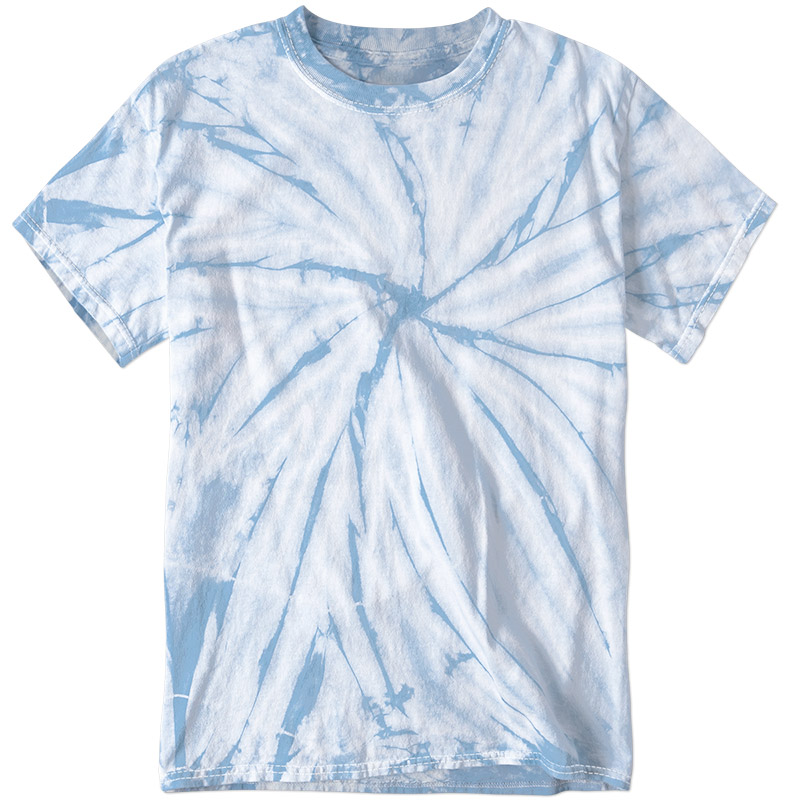This image features a half-sleeve, round-neck t-shirt prominently displayed against a white background. The t-shirt showcases a tie-dye design in varying shades of blue and white. The intricate pattern resembles star-shaped waves radiating from the center, with blue projections extending outward. The design covers the entire t-shirt, including the sleeves and neck area, and notably, there are no logos or text on the garment. Although the t-shirt is predominantly white with light blue tie-dye, certain areas, such as the collar, lower left, and sleeves, exhibit a higher concentration of darker blue, providing a rich contrast and depth to the pattern. Overall, it is a simple yet visually striking piece, likely designed for males.